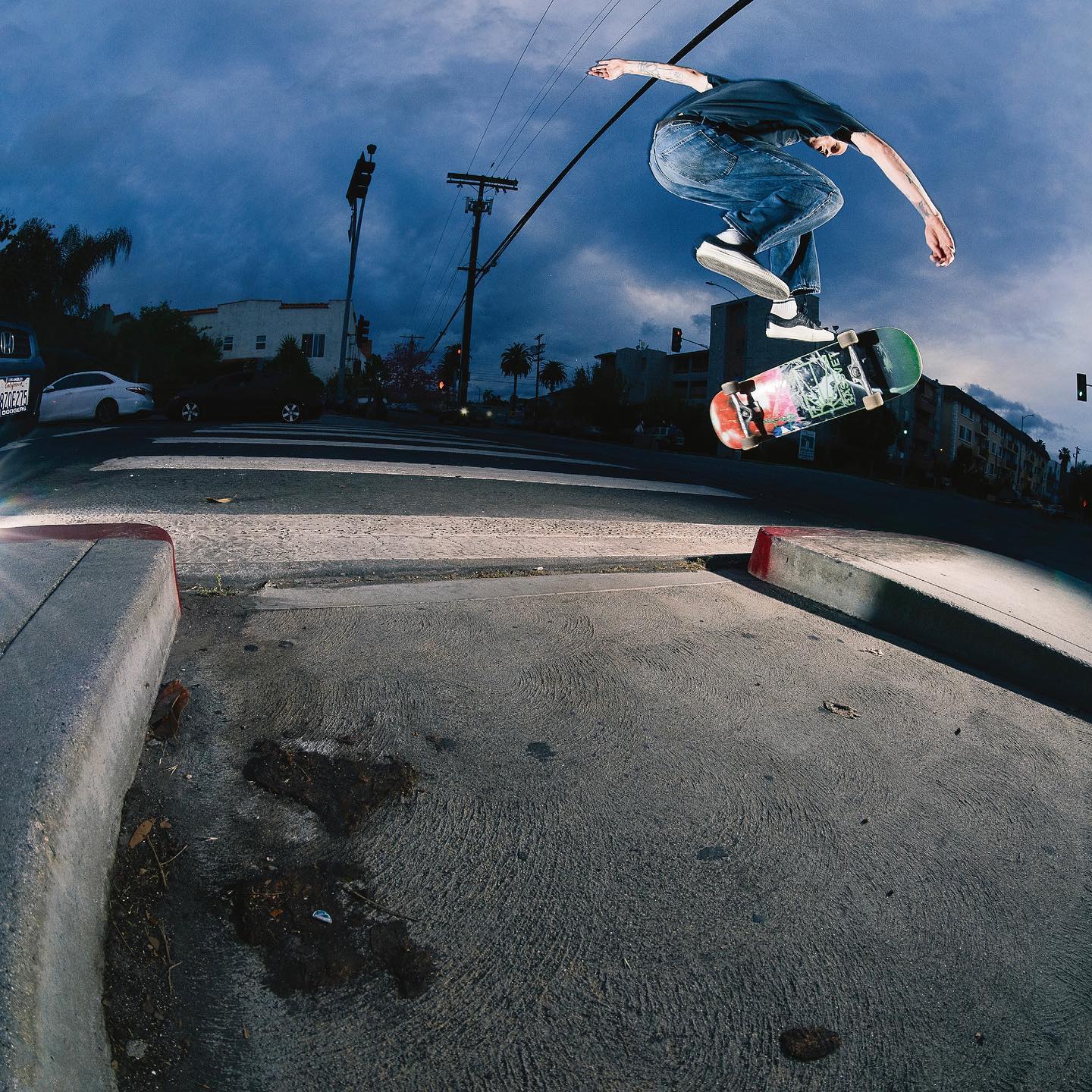This image beautifully captures a dramatic moment of skateboarding action set against a dusky Southern California backdrop. The perfectly square photo is divided into three horizontal sections: the top third is dominated by a dark, cloud-covered evening sky that hints at impending nightfall. Below, architectural features like wire poles, trees, various buildings, and a street come into view, complemented by a car and a distinct California license plate, hinting at the location.

In the central and lower sections, a concrete asphalt street flanked by two sidewalks is visible. The most striking element, however, is the skateboarder soaring through the air in the upper right quadrant of the image. The skateboarder, a Caucasian male dressed in a short-sleeved navy blue t-shirt, blue jeans, and white sneakers with white socks, is captured mid-kickflip. His arms are extended—his right arm thrust forward and his left arm trailing behind him—as he attempts to control the board beneath him. The skateboard, suspended just below his feet, has cream or grayish wheels and a decorated underside in shades of red and green, flashing glimpses of its dynamic design. The scene is rich in detail, from the clothing and posture of the skateboarder to the surrounding urban and natural landscape, collectively evoking the vibrant yet tranquil spirit of a Southern Californian evening.